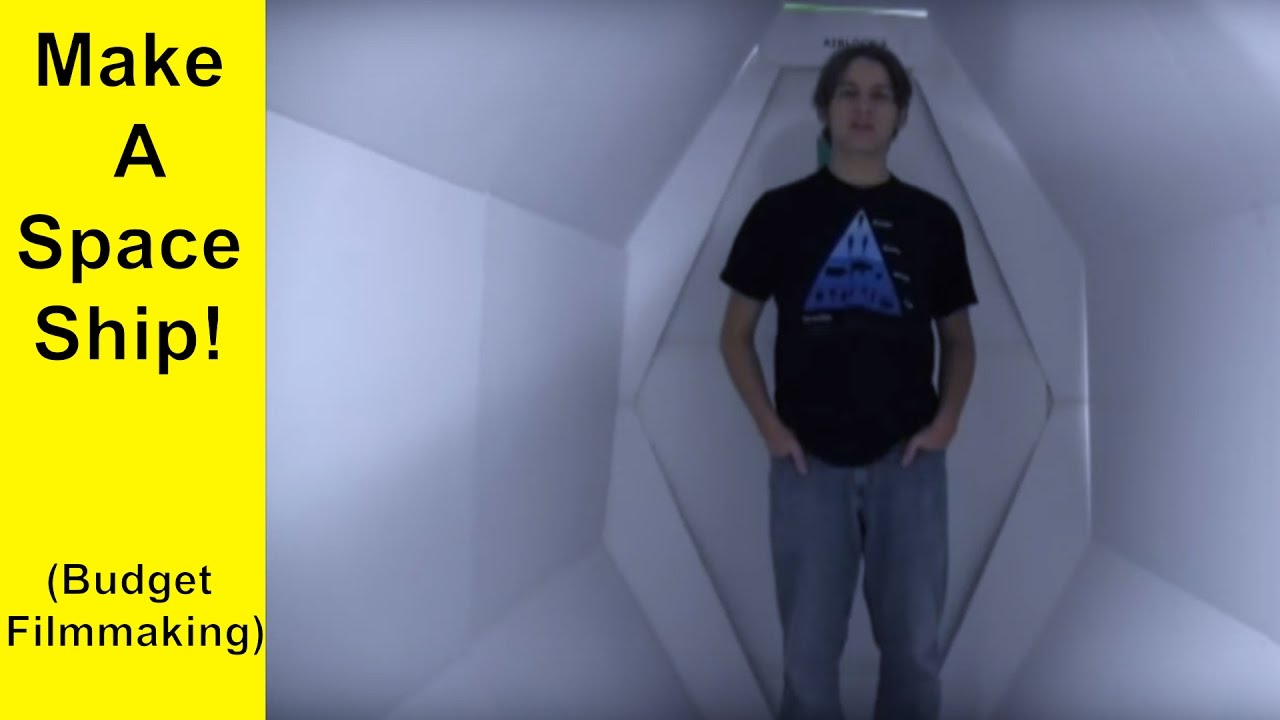In the image, a young man or teenager is standing inside a makeshift spaceship or pod, constructed from white materials that resemble thin cardboard or paper. The interior appears futuristic yet homemade, designed to mimic a spaceship without the expense of a large set. The room is low-lit, enhancing the space-themed ambiance. The young man is wearing a black graphic t-shirt featuring a blue pyramid design, along with blue jeans. His hands are tucked into his pockets, and he is looking directly at the camera, not speaking. On the left side of the image, there is a yellow rectangle with the text "Make a Spaceship" in large font and "Budget Filmmaking" in smaller font within parentheses, suggesting the image is a YouTube thumbnail for a video about creating a budget-friendly spaceship set for filmmaking.